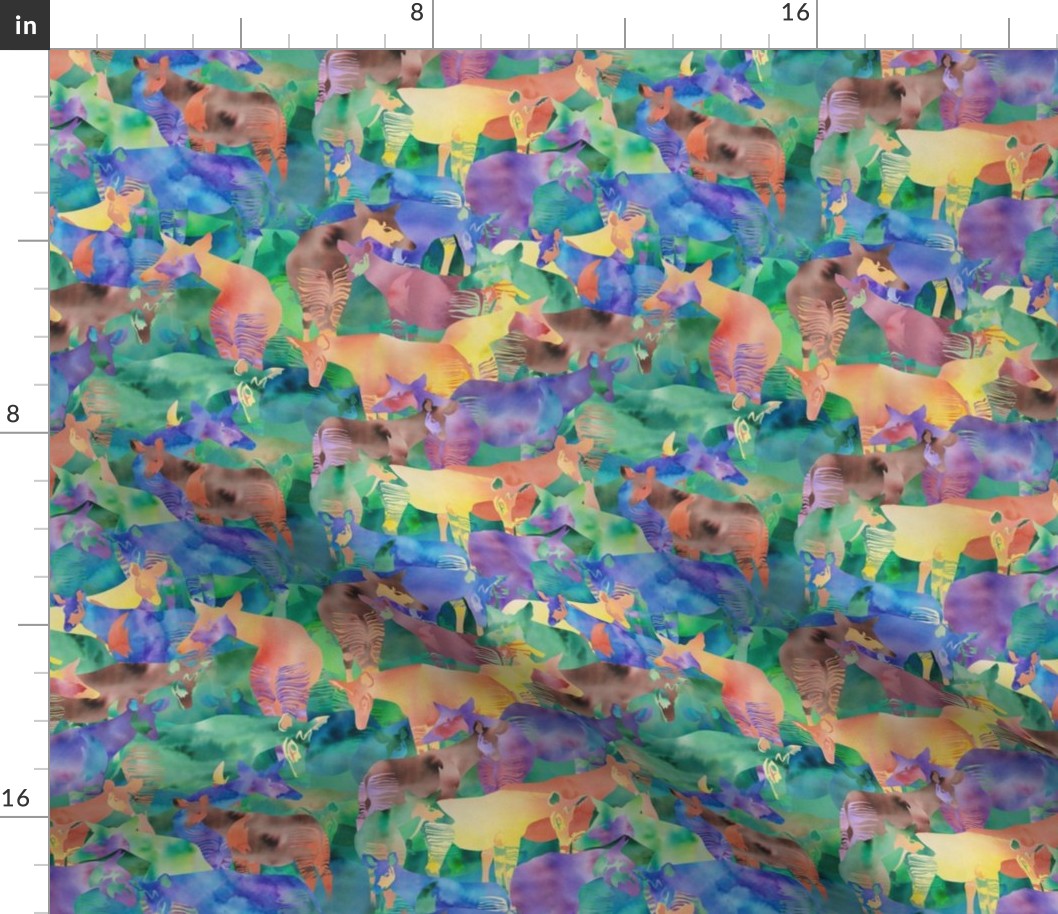The image depicts a vibrant tapestry, measuring approximately 18 by 21 inches, adorned with a mesmerizing array of colors including green, blue, purple, yellow, orange, red, pink, and brown. The background hues blend seamlessly while maintaining distinct borders around the featured animals, likely African antelopes, identifiable by their uniquely patterned hind legs. The artistic style resembles watercolor, creating a repeating pattern of various animals such as deer, zebras, and giraffes, each distinguished by its own set of colors. The tapestry includes a scale along the top and left edges, indicating inches, suggestive of its use as both decorative art and a potential growth chart. Suitable for children’s decor due to its playful and whimsical design, the detailed craftsmanship and rich color palette ensure that it remains equally appealing to adults.